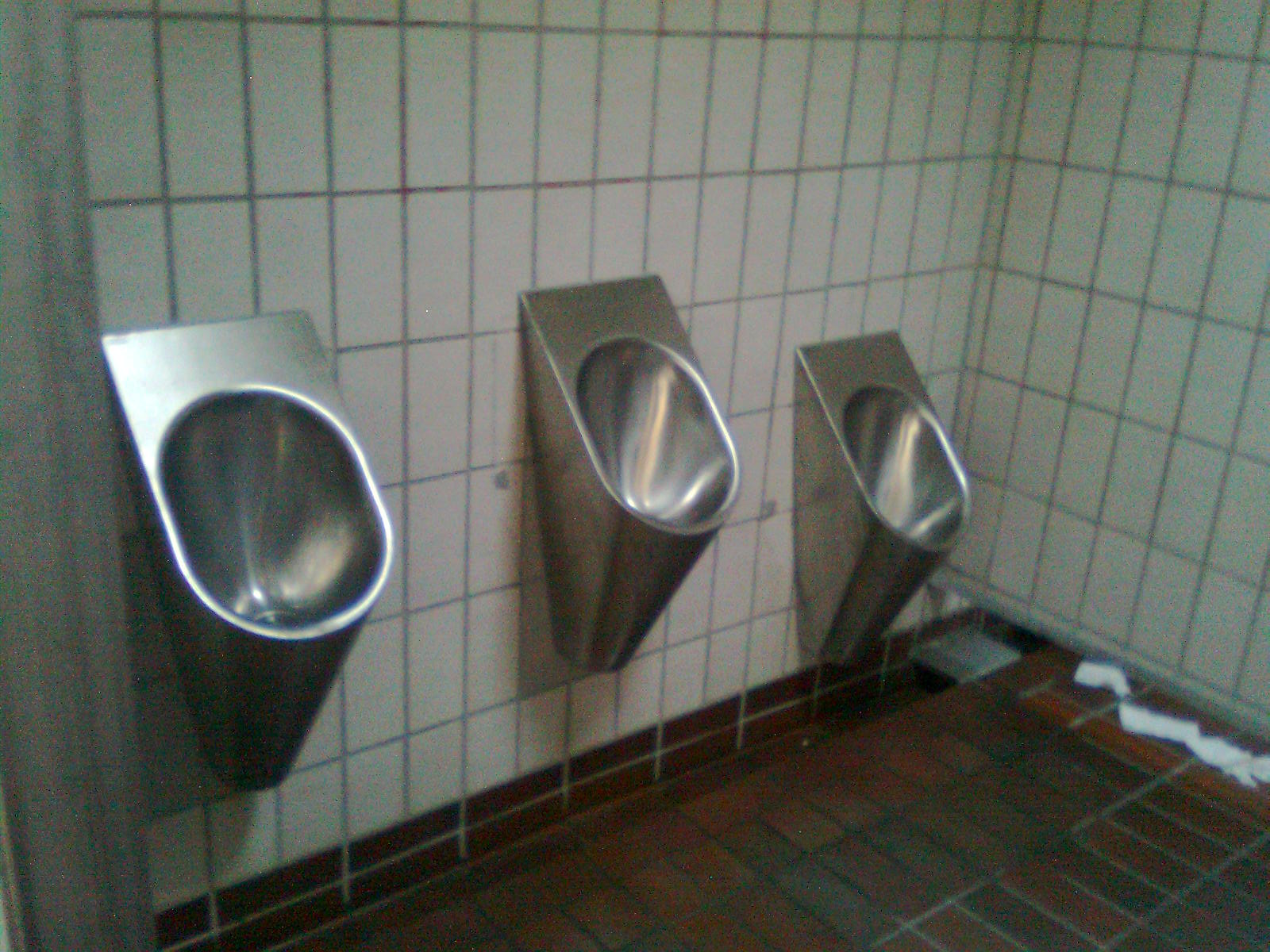This color photograph, slightly dark and a bit out of focus, captures a corner of a men's bathroom. The horizontal, rectangular image showcases three stainless steel, conical-shaped urinals mounted on a wall of large white tiles that appear somewhat grimy. Two urinals are aligned at a standard height, while the third, nearest the corner, is positioned lower. The urinals feature a minimalist design with no flush handles, just open holes at the bottom leading into a tiled trough. The trough and the worn floor are made of red tiles, with a dark, grimy hue noticeable near the urinals. A brown tile border runs along the base of the wall. On the right side of the image, against a perpendicular wall, pieces of wet toilet paper are scattered near a gray drain. The scene reflects a utilitarian and somewhat neglected restroom environment.